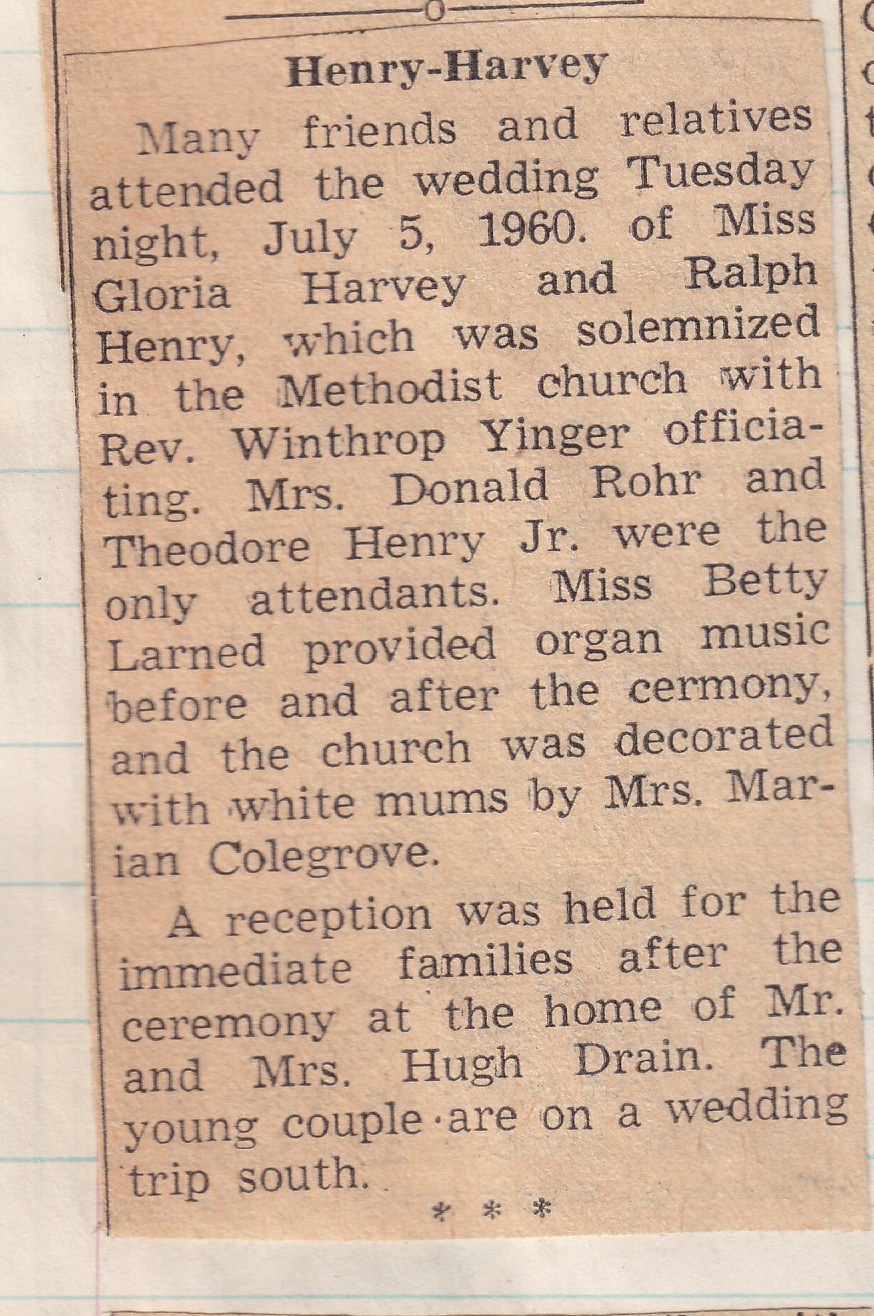This photograph features an aged, yellowed newspaper article cut and pasted onto lined notebook paper. The headline reads "Henry-Harvey." The article details the wedding of Miss Gloria Harvey and Ralph Henry, which took place on Tuesday night, July 5, 1960, at the Methodist Church with Reverend Winthrop Yinger officiating. Mrs. Donald Rohr and Theodore Henry Jr. attended the couple, while Miss Betty Larned provided organ music before and after the ceremony. The church was decorated with white mums by Mrs. Marion Colgrove. Following the ceremony, a reception was held for immediate family at the home of Mr. and Mrs. Hugh Drain. The newlyweds embarked on a wedding trip to the south.